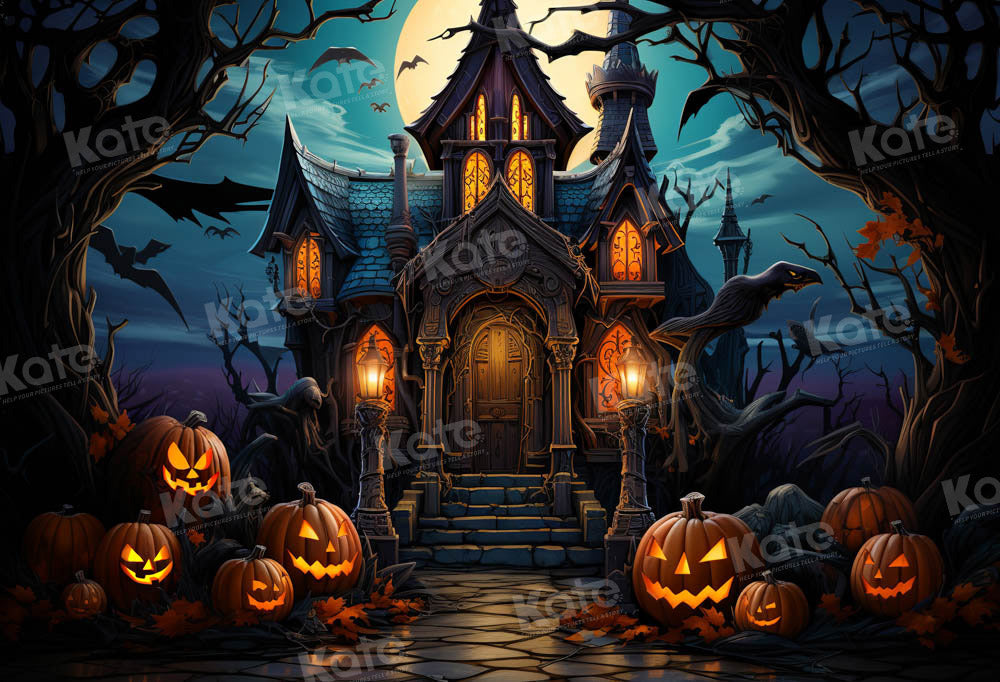The image is a detailed cartoon-style painting of a spooky haunted mansion, predominantly featuring neutral gray colors. The house has a blue-tiled roof and is fronted by wooden doors and columns adorned with lanterns. Gray stones form a path leading to the entrance. The windows are illuminated, casting an eerie glow. Surrounding the mansion are numerous orange jack-o'-lanterns with smiling, leering faces, positioned on either side of the house next to nearly barren trees with sparse orange leaves. The night sky is a dark blue with a full yellow moon partially obscured by clouds, and there are black bats and possibly an owl or crow flying around. The image has white watermarks with the name "Kate" on them, though some text remains indistinguishable.